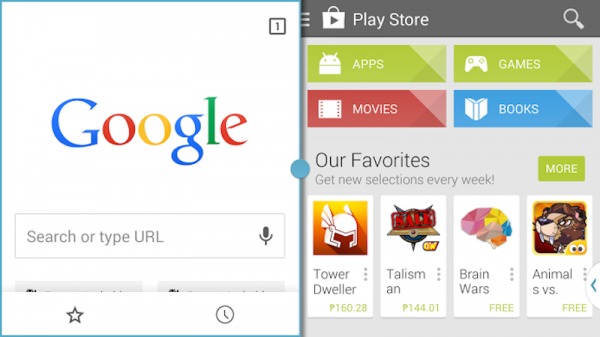Here is the revised and detailed caption:

---

This is a detailed screenshot depicting elements from both Google and the Google Play Store, arranged in a split-screen style. On the left side of the screen, the standard Google logo is prominently displayed in its iconic colors: a blue capital 'G,' followed by a lowercased red 'o,' yellow 'o,' blue 'g,' green 'l,' and red 'e.' Beneath the logo is a search bar labeled "search or type URL," accompanied by a microphone icon for voice input. Below the search bar, there are two buttons, but their text is partially cut off. In the bottom left-hand corner of this section, there is a star icon, while the bottom right-hand corner features a clock icon. In the upper right-hand corner, a small box displaying the number '1' can be seen.

The right side of the screen is partially cut off but reveals elements of the Google Play Store. It contains a search bar labeled "Play Store," which includes a magnifying glass icon denoting the search function. Below the search bar are two prominent green bars: one labeled "Apps" with an Android symbol, and the other labeled "Games" with a controller icon. Underneath, there is a red button labeled "Movies" featuring a filmstrip icon, followed by a blue section labeled "Books" with a white book icon.

---

This detailed caption provides a clear and comprehensive description of the screenshot, outlining all visible elements and their positions.